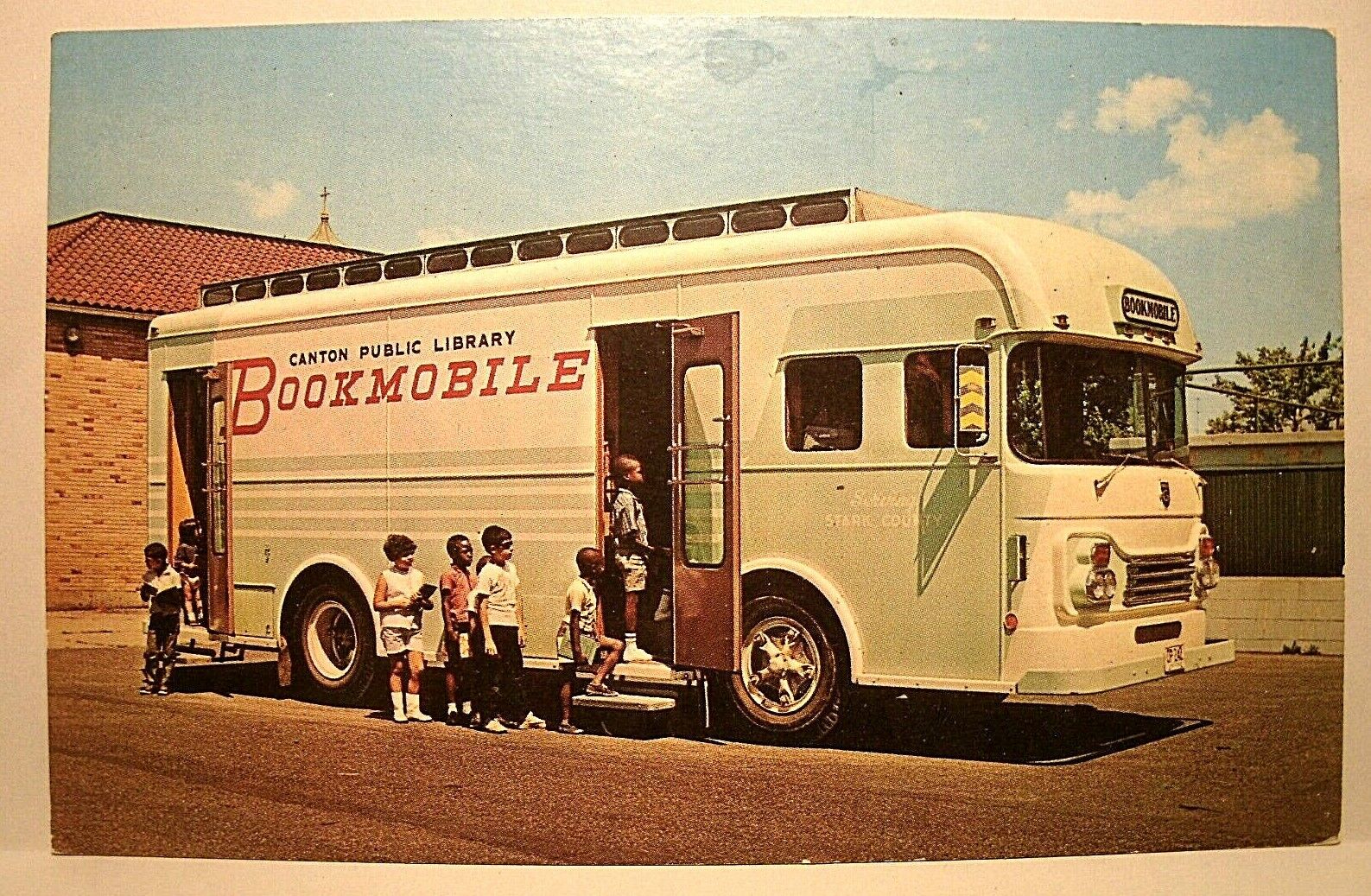This vintage photograph from the 1950s or 60s captures a sunny day with a vibrant blue sky. The photo, mounted on a cardboard backing visible around all four edges, features the Canton Public Library Bookmobile, a large bus-like vehicle with a faded green and white exterior. Centered in the image, the bookmobile has two open doors—one near the back and one behind the front tire. From door to door, "Canton Public Library" is inscribed in black at the top, with "BOOKMOBILE" in red capital letters below it. Additionally, "BOOKMOBILE" is written above the windshield.

A group of eager young children, possibly six or seven years old, forms a line waiting to enter the bookmobile. Some kids are holding books, and one child is seen exiting through the back door. In the backdrop, there is a complex landscape: a concrete building, a wooden fence, a cinder block wall, and a brick structure with orange and brown hues and a yellow tiled roof, possibly resembling a church with a visible cross. The greenery includes trees to the right of the image. The scene is set either on a grassy area or a parking lot, emphasizing the community's engagement with this nostalgic mobile library service.